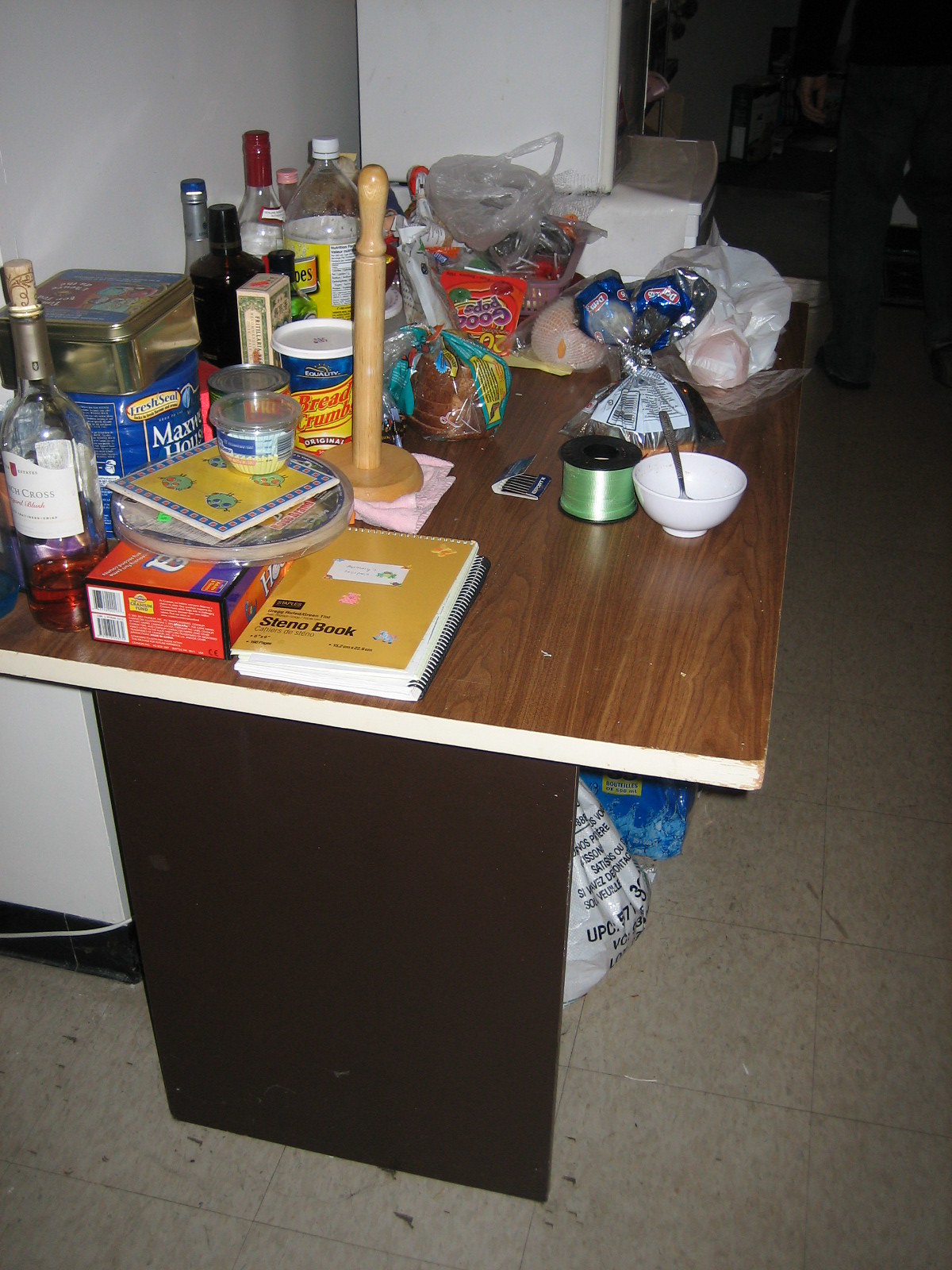This photograph captures a cluttered table in what appears to be a break room, its nondescript environment reminiscent of an elementary or high school setting, characterized by heavily scuffed tiles. The table itself is simple, featuring side panels and a thick faux wood grain laminate tabletop edged in white, with noticeable wear and tear on the corners. 

The table is laden with a miscellany of items: a wooden paper towel roll holder, several almost-empty bottles of alcohol, including a bottle of wine, and a bottle of Schweppes tonic water. Scattered paper plates wrapped in plastic, a steno notebook with a ring binder, a book of matches, and potential candy or balloons add to the disarray. There are breadcrumbs, cupcake paper holders, child-themed party napkins, a can of Maxwell House coffee, and more bottles of alcohol lurking in the background. Additional clutter includes numerous plastic bags, possibly filled with trash or fruit, an empty bowl with a spoon, and a few plastic trays.

A person in jeans and a long-sleeved black T-shirt stands in the upper right-hand corner, facing away from the camera, further highlighting the focal point on the table. This scene conveys an atmosphere of either the aftermath of a festive gathering or a very disordered break room in an office.